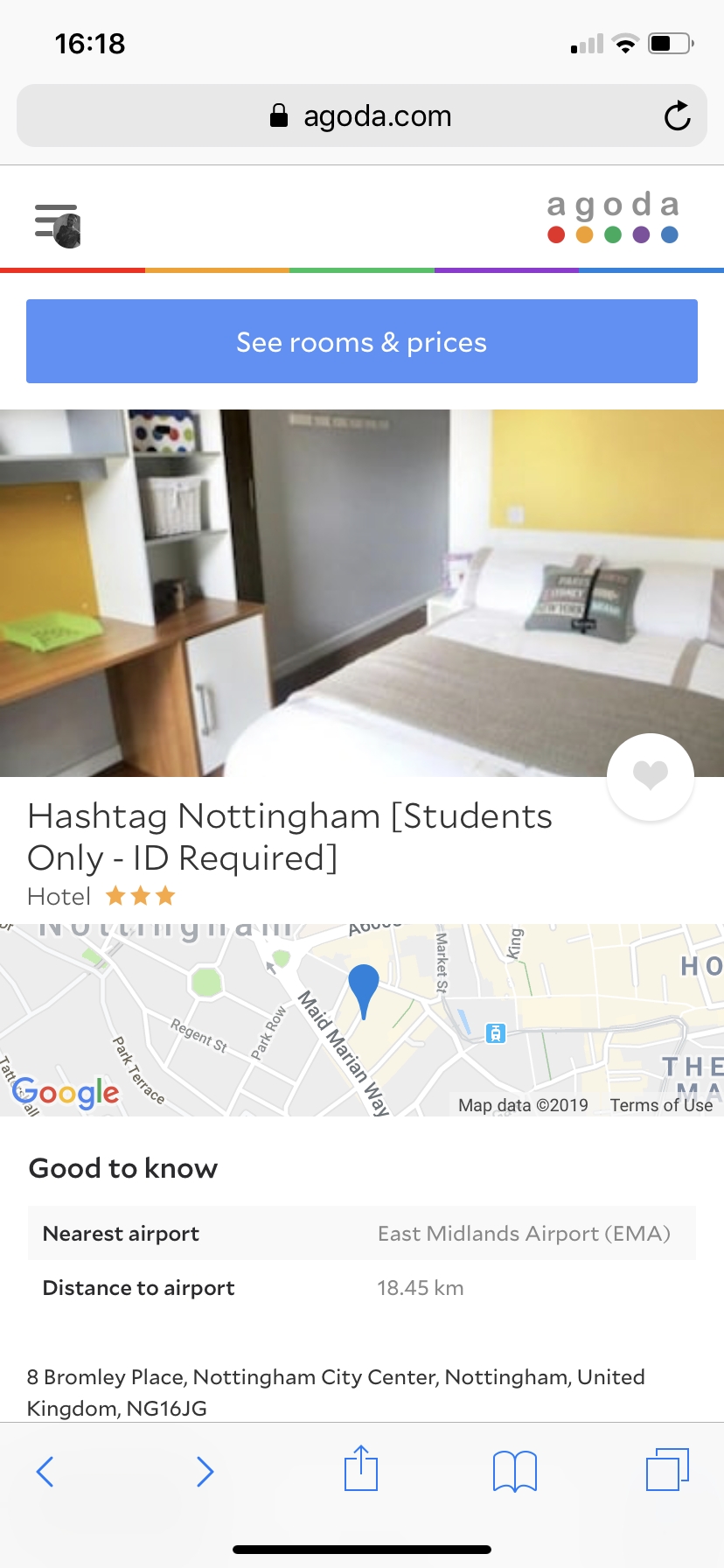This image depicts a screenshot taken from a cell phone displaying the Agoda.com interface. At the top of the screen, the Agoda logo is prominently featured, accompanied by colored dots in red, orange, green, purple, and blue. Below this, there is a photograph that appears to be of a bedroom, likely representing a lodging option.

The text below the image includes the hashtag "Nottingham students only ID required," indicating that the accommodation is exclusively available to students in Nottingham. The listing is categorized as a hotel with a three-star rating, as shown by the three filled stars next to it.

At the very top of the screen, a blue rectangular button labeled "See rooms and prices" invites users to explore further options. Below the bedroom image, there is a section with a map pinpointing the location of the accommodation, with the word "Google" written within this segment. Under the map, information is provided under the "Good to know" section, listing details such as the nearest airport and the distance to the airport. At the bottom of the screen, there are several clickable icons offering additional features or options related to the listing.